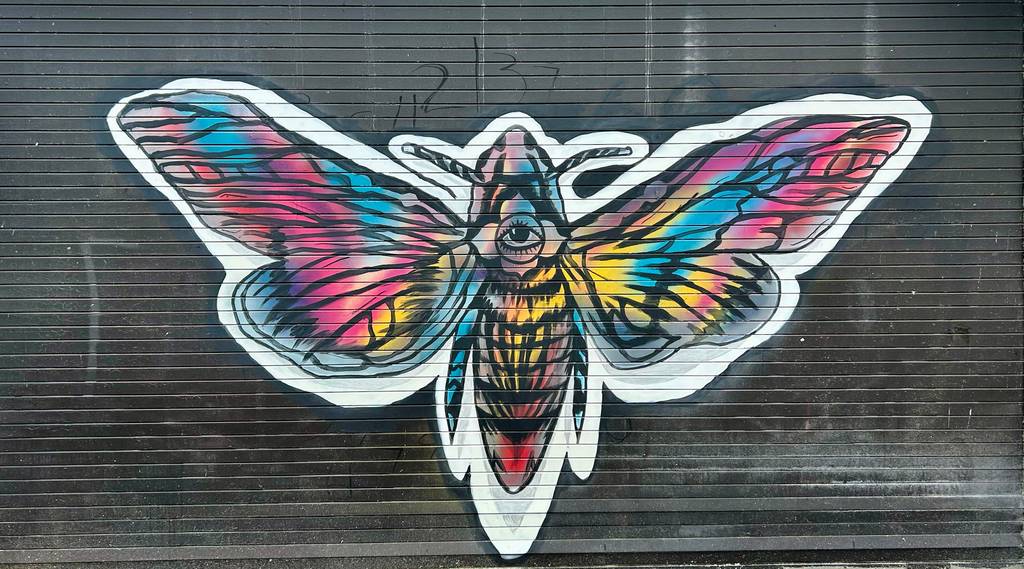The image showcases a vivid graffiti painting of a butterfly or moth on a black roll-top door, likely situated beside a sidewalk. The butterfly's wings are adorned with a spectrum of colors including red, blue, yellow, pink, and purple, and are outlined in white. Each wing reveals a unique blend of these vibrant hues, giving the creature a rainbow-like appearance. Prominently featured on the center back of the butterfly is a black, human-looking eye. The butterfly also sports two visible legs and antennas. The surface of the door has horizontal lines and a slight reflection, adding texture to the scene. There is also numbered text above the butterfly, enhancing the urban artistic vibe.